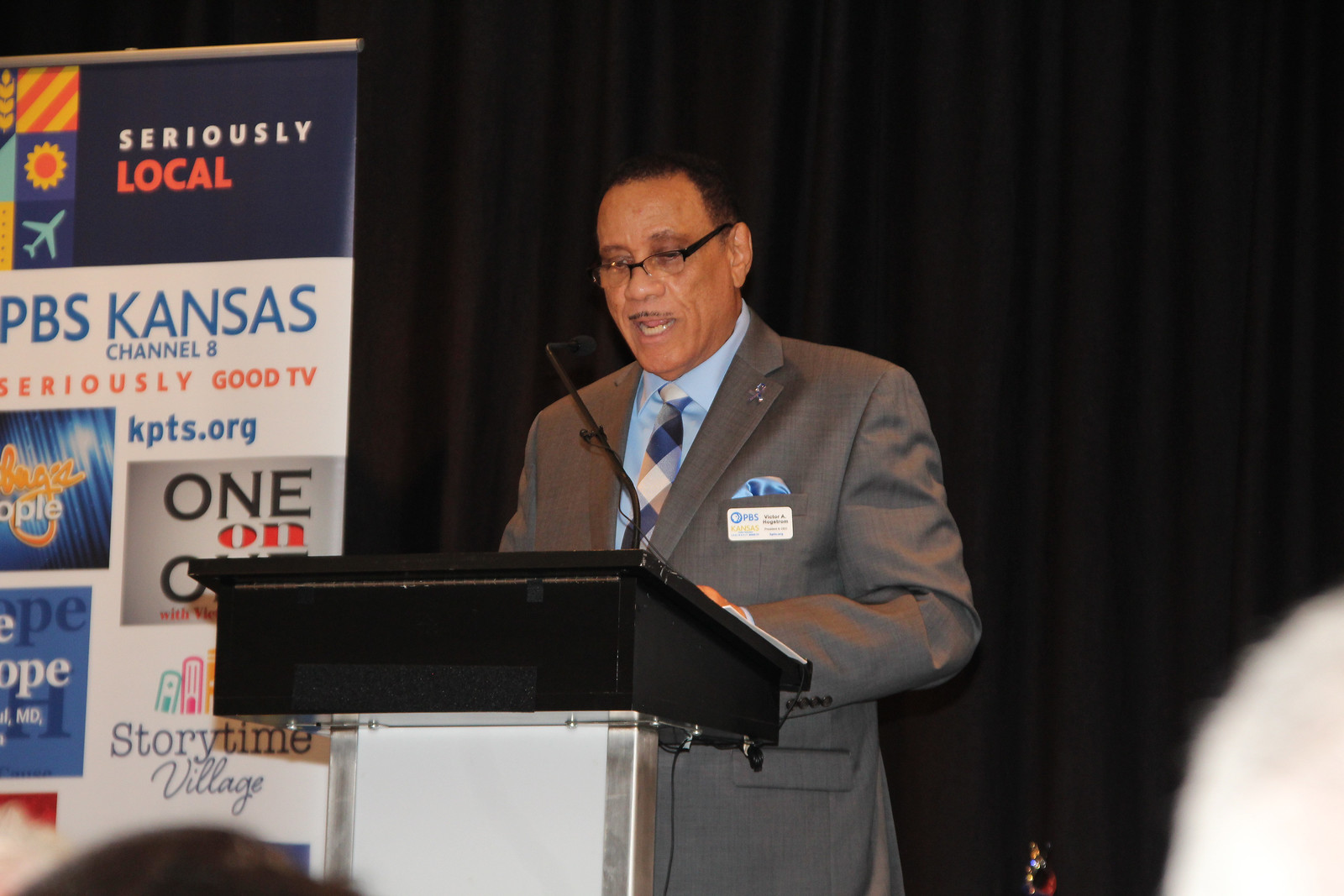This photograph captures an African-American man delivering a speech at a black podium. He's equipped with a small microphone near his face and is reading from a document placed on the podium, which is partially obscured. The man has dark skin, very short, cropped dark hair, a thin mustache, and glasses with black frames. He is dressed in a medium gray suit, a light blue dress shirt, and a multicolored tie featuring shades of blue, white, and orange. A light blue pocket square and a name tag are also visible on his suit. The background features a very dark, almost black curtain, while to his left, there is a large board with multiple logos and text. It prominently displays "Seriously Local, PBS Kansas, Channel 8, Seriously Good TV, KPTS.org" at the top, with some words partially cut off, and "Storytime Village" at the bottom, set against a white backdrop with blue and orange text.